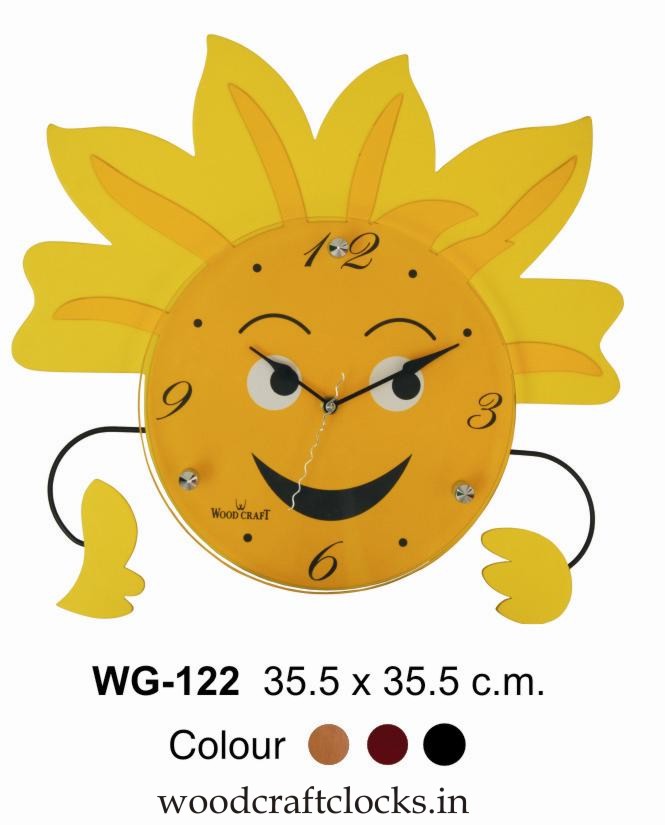The image portrays a whimsical circular clock designed to look like a cheerful sun. The bright yellow clock face features a smiling expression with vividly detailed black and white eyes and expressive eyebrows. The hours 12, 3, 6, and 9 are clearly marked, while the other hours are indicated by small dots. The clock hands resemble playful, spindly black arms with yellow pads on the tips, and they point to a time of approximately 10:10. Extending from the top portion of the clock are bright yellow sunbeams, enhancing its sunny appearance. Below the clock face, it displays the model number WG122 and its dimensions of 35.5 by 35.5 centimeters. The clock is available in three different colors: brown, red, and black. It is manufactured by woodcraftclocks.in.